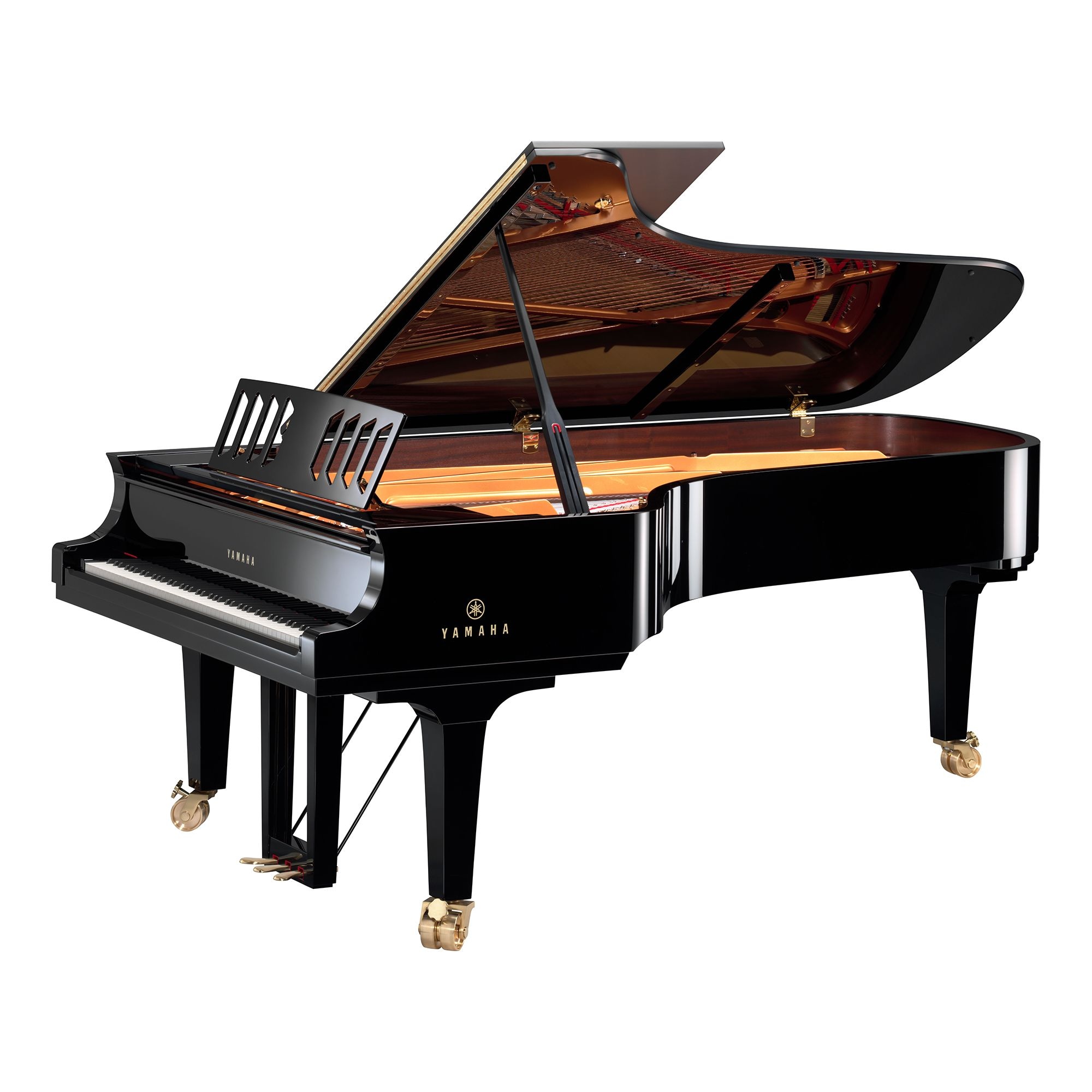This image showcases a Yamaha Grand Piano with meticulous details and a sense of luxurious craftsmanship. The piano stands predominantly in a glossy, dark brown, almost black finish that gleams under the light, exuding an air of elegance and professionalism. It's positioned on a plain white background that accentuates its refined design. Visible from a side view, the piano is open, with its lid propped up by a support, revealing an interior awash in an orangey-yellow hue, in stark contrast to the exterior, hinting at the high-quality construction.

The left side of the piano prominently features the classic white and black keys, and directly above them, there's a sophisticated logo clearly marking it as a Yamaha. The stand above the keyboard, elaborately designed with hollowed patterns and eight openings, serves as the holder for music scores. The piano rests on three legs, two on the left and one tapered on the right, each fitted with polished brass rollers, adding to the piano's mobility and luxurious appearance.

At the bottom, three gold-colored foot pedals are visible, hinting at the potential for a rich and dynamic range of musical expression. The overall dimensions suggest a substantial presence, estimated to be around nine feet in size, confirming its status as a professional-grade instrument likely to be found in a concert hall or a high-end music studio.